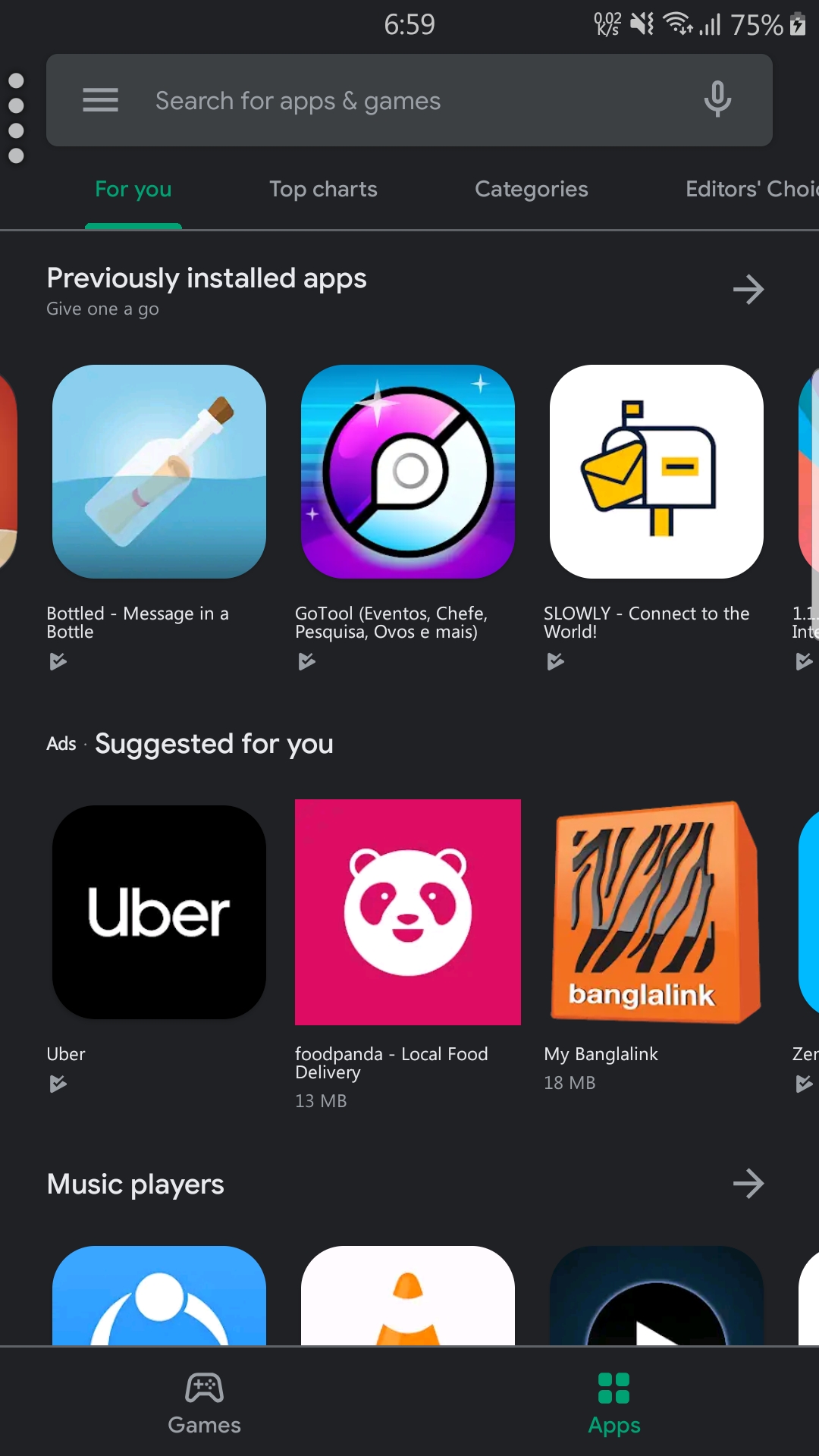This screenshot, taken from a cell phone, captures the App Store interface at precisely 6:59, as indicated by the time displayed at the top bar. The top-right corner showcases the phone's status icons: muted volume, an active Wi-Fi connection, cellular service signal, and a battery level at 75%, represented by a battery icon.

Beneath these indicators lies a search bar designed for users to search for apps and games. To the left of the search bar, three horizontal lines enable further filtration by categories, while on the right, a microphone icon allows for voice input.

Below the search bar, a navigational menu appears with tabs labeled: "For You," "Top Charts," "Categories," and "Editor's Choice." This is followed by a section titled "Previously Installed Apps," featuring a clickable arrow for viewing a detailed list of apps that were previously installed on the device.

Next, there's a section labeled "Ads Suggested for You," displaying personalized app suggestions for the user. Further down, the category "Music Players" is featured with an additional arrow to explore more music-related apps.

Finally, at the bottom of the screen, there are two navigation tabs: "Games" on the left and "Apps" on the right, with the latter being selected as evident in this screenshot.